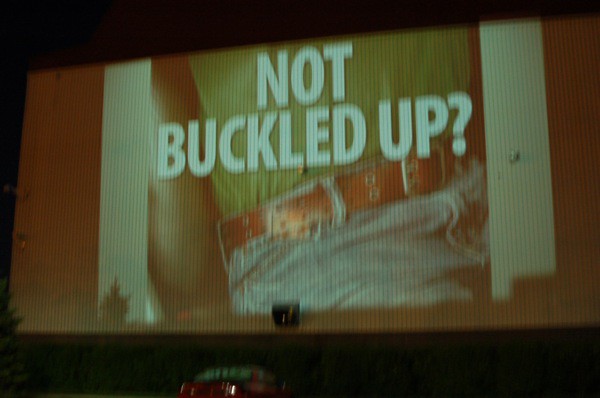The photograph captures a nostalgic drive-in movie theater scene at dusk. Dominating the image is the large drive-in screen, displaying a public service advertisement. The ad features the torso of a person dressed in a green shirt and blue jeans, accessorized with a brown belt, accompanied by the bold white text: "Not Buckled Up." Distinct two white lines run vertically on either side of this central image, framing the ad. Below the visual, a small, black, square object appears to be mounted on the screen structure.

At the bottom of the photo, a red car is partially visible, adding a touch of vibrancy to the scene. Framing the sides of the screen are dark, rectangle shapes, likely structural elements of the setup. In the background, a line of trees creates a natural border, their shadow casting a distinct silhouette on the lower part of the screen. The scene captures the serene ambiance of an evening at a drive-in, blending elements of nostalgia with a modern safety message.